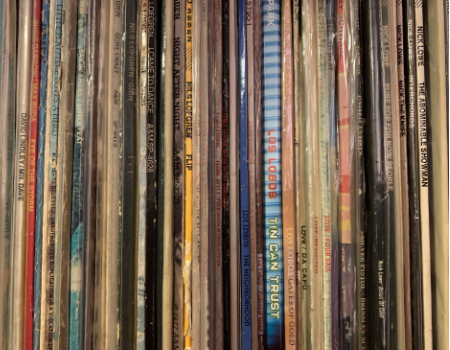This color photograph captures a tightly packed row of approximately 20 to 30 old LP records, displayed upright on a shelf that is not visible due to the close-up framing of the image. The albums, many of which are weathered and faded, fill the entire frame from top to bottom and left to right, creating a feeling of claustrophobia. Some of the record spines are wider, suggesting gatefold sleeves, while others are thinner. A few are wrapped in plastic film, though most are not. Damage is evident on some of the spines, with visible splits and cracks in the jackets. The album titles, while hard to read, include "Nick Lowe: The Abominable Showman" and "Los Lobos: Tin Can Trust," with the latter featuring noticeable light and dark blue stripes. Despite a mix of colors, the overall scene remains subdued, with various shades of fading contributing to the vintage aesthetic.